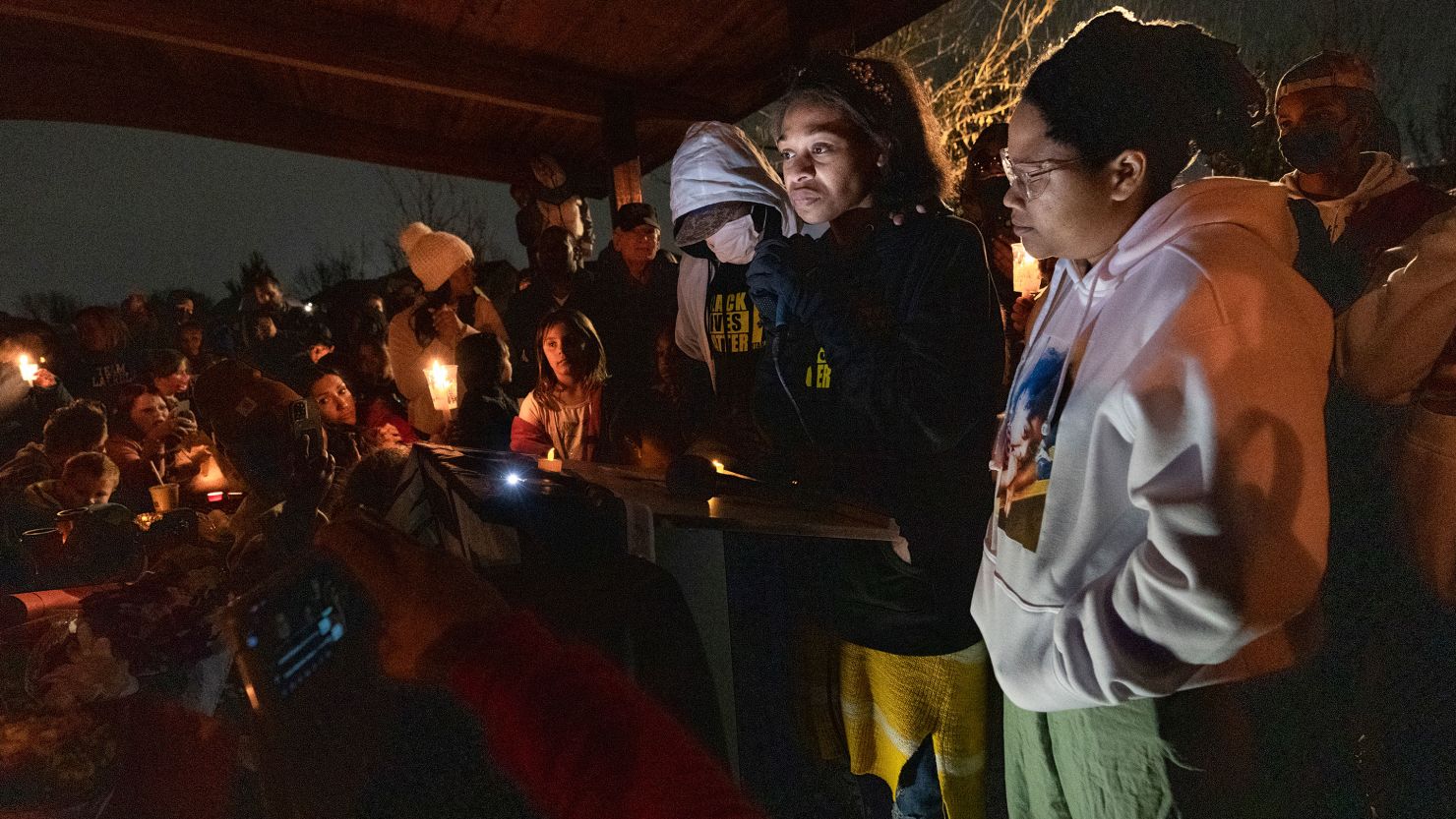The image depicts a nighttime gathering under an outdoor, wooden-roofed gazebo or shaded area, providing shelter without walls. The scene appears to be somber, potentially a vigil or a memorial event, as indicated by the serious expressions and the possible holding of lights or candles in cups by some attendees. The cold weather is evident, with everyone donning jackets, sweatshirts, long pants, and even gloves, along with some wearing face masks. Prominently, on the right side of the image, a black-skinned woman stands at a lectern, holding a microphone, likely delivering a speech. She is somewhat illuminated, her face grave and reflective, next to another black-skinned woman with glasses. Behind them, a masked man can be seen, along with another hooded and masked individual, hinting at potential COVID-19 precautions. The overall atmosphere is dark, possibly overcast, with the open-air structure offering limited protection against the cold night.